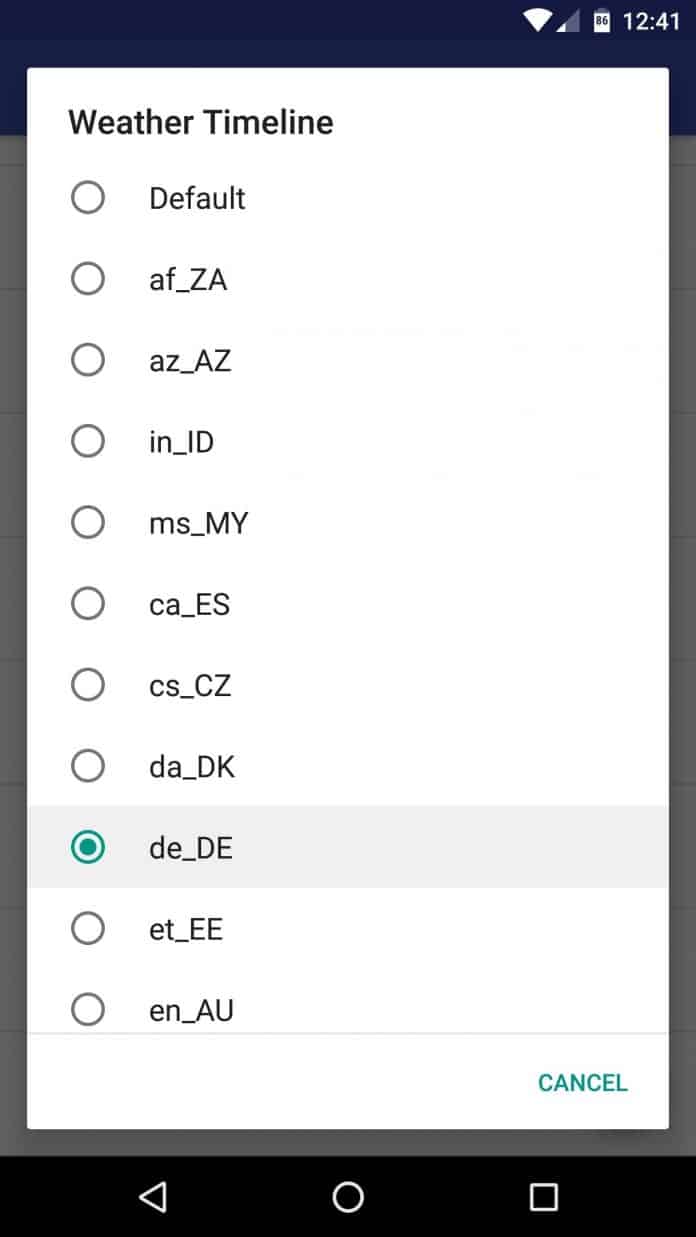This image displays a detailed weather timeline interface where users can select different countries via a series of clickable buttons. At the top, the default option is highlighted. Below, various country codes are listed in uppercase format, including "AF_ZA," "AZ_AZ" (possibly Azerbaijan), "IN_ID," "MS_MY," "CA_ES," "CS_CZ," "DA_DK," "DE_DE" (likely Deutschland or Germany). The currently selected country is "DE_DE," indicating the user is viewing weather information for Germany. Additional options such as "ETE" and "ENAU" (likely representing Australia) suggest a wide array of country choices. Recognizable country codes like "CS_CZ" for Czechoslovakia, and "CA_ES" for Spain, are also present. This detailed selection interface indicates potential weather data availability for numerous international locations.